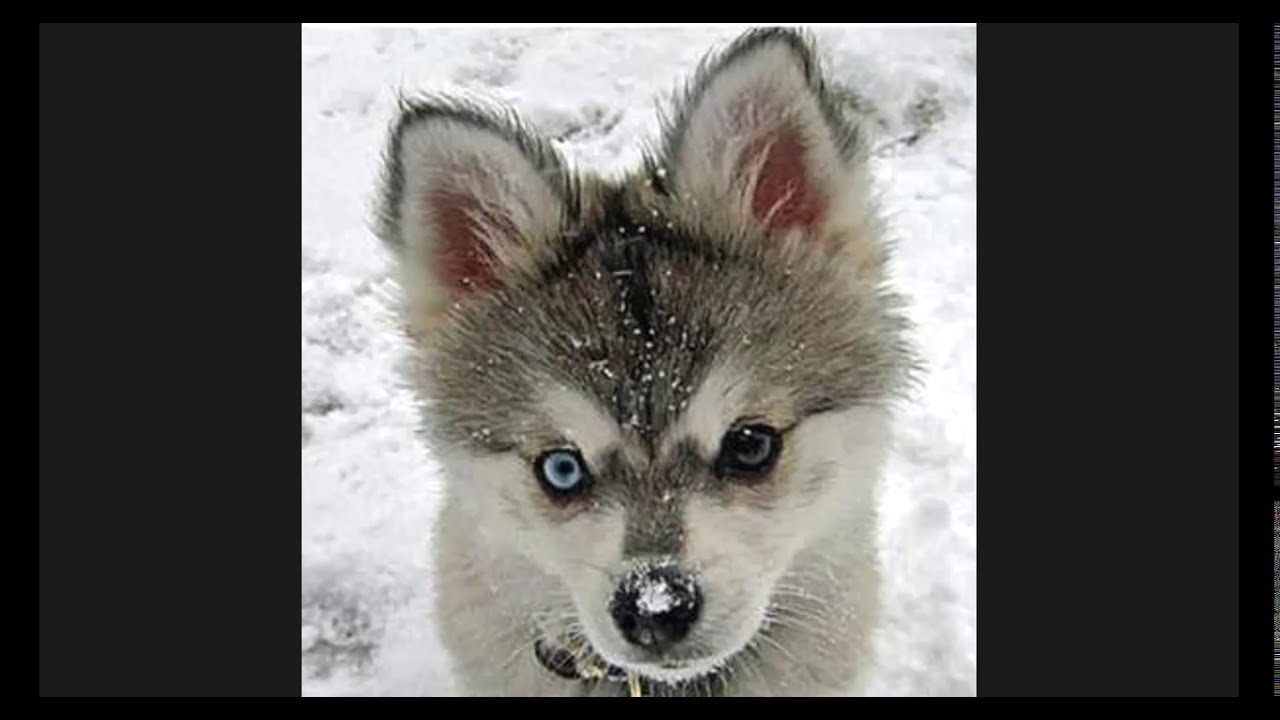In this detailed image, we see a very small Siberian Husky or Malamute puppy, standing outdoors in a snowy environment. The puppy is positioned directly in the center of the image, facing the camera with his furry ears pointed straight up. The background is a snowy yard, suggesting an outdoor setting possibly during a snowstorm.

The puppy's striking features include piercing blue eyes, with one eye slightly darker than the other, and a black nose dusted with snow, adding to his wintry appearance. The top of his head is mostly dark fur, contrasting with the white fur above his eyes and around his face. His face is predominantly white, extending down to his neck, which is partly obscured by his fur. He also seems to be wearing a collar, although it's mostly hidden beneath his thick fur.

The color palette of the image is quite varied, with shades of black, gray, white, light blue, and pink visible in the puppy's fur and the snowy background. His adorable, inquisitive expression is captivating, as he gazes directly into the camera, making for a charming and memorable photograph.